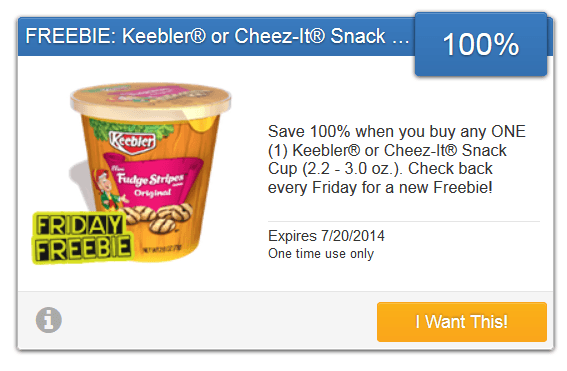The image is a rectangular advertisement with a prominent horizontal layout. At the top, there is a blue banner with white text that reads, "Freebie: Kirby® or Keebler® or Cheez-Its® Snack..." followed by "100". In the upper right corner of the blue banner, there's a small blue rectangle containing "100%" in white text.

Below the banner, there's a photograph of a Keebler Fudge Stripes Cookies snack cup, resembling a cup of soup. The snack cup has a lid and is adorned with a colorful design featuring red, brown, light brown, golden brown, white, and green elements. Text on the cup reads, "Save 100% when you buy any one Keebler or Cheez-It snack cup. 2.2-3.0 ounces". Additional information indicates, "Check back every Friday for a new freebie. Expires 7-20-2014. One time use only."

In the top left of the cup, there's a label featuring "Freebie Friday" written in yellow letters on black squares, with the black squares outlined in yellow.

Finally, at the bottom right corner of the advertisement, there is an orange button with white text stating, "I want this".